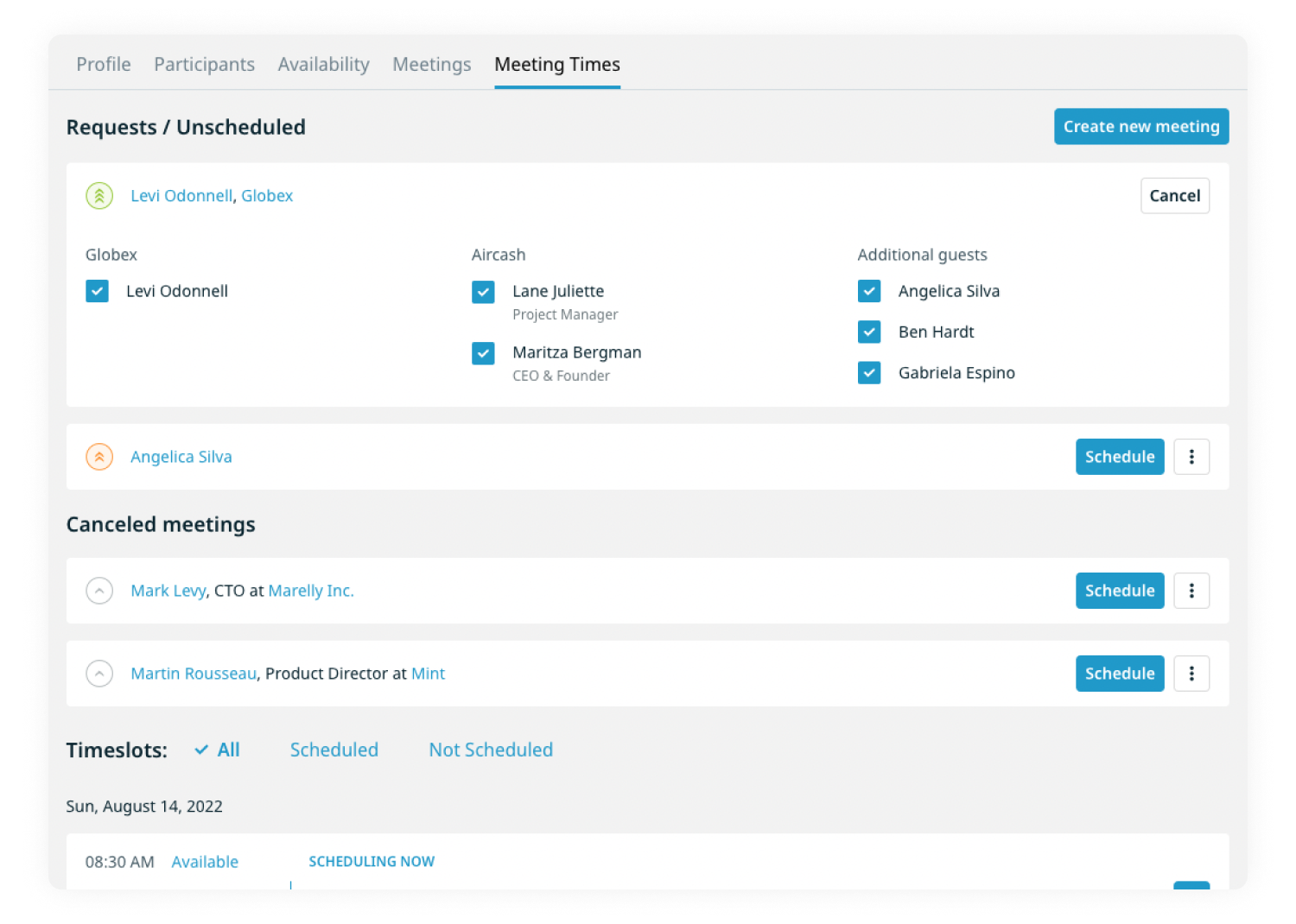This screenshot, taken from a predominantly gray and white themed website, showcases the "Meeting Times" page, which is the currently selected section as indicated by its bolded text and the blue underline. The website's top navigation bar displays options from left to right: Profile, Participants, Availability, Meetings, and Meeting Times. 

Beneath the "Meeting Times" header, the section is subdivided into categories. The first category, labeled "Request/Unscheduled," features entries such as "Levi O'Donnell, Globex," with "Globex" followed by a blue box containing a white checkmark and the name "Levi O'Donnell." 

In the center, under the heading "Air Crash," and on the right, under "Additional Guests," there are names listed in respective columns, indicating participants and guests for various meetings. 

Further down the page, a bolded heading "Cancelled Meetings" is followed by yet another bolded heading "Time Slots." The page also lists a specific date, "Sunday, August 14th, 2022," near the bottom, suggesting available or previous meeting dates. On the far right side, a prominent blue box with the text "Create New Meeting" stands ready for users to schedule new meetings. The page layout allows users to manage their meetings and view participant details efficiently.